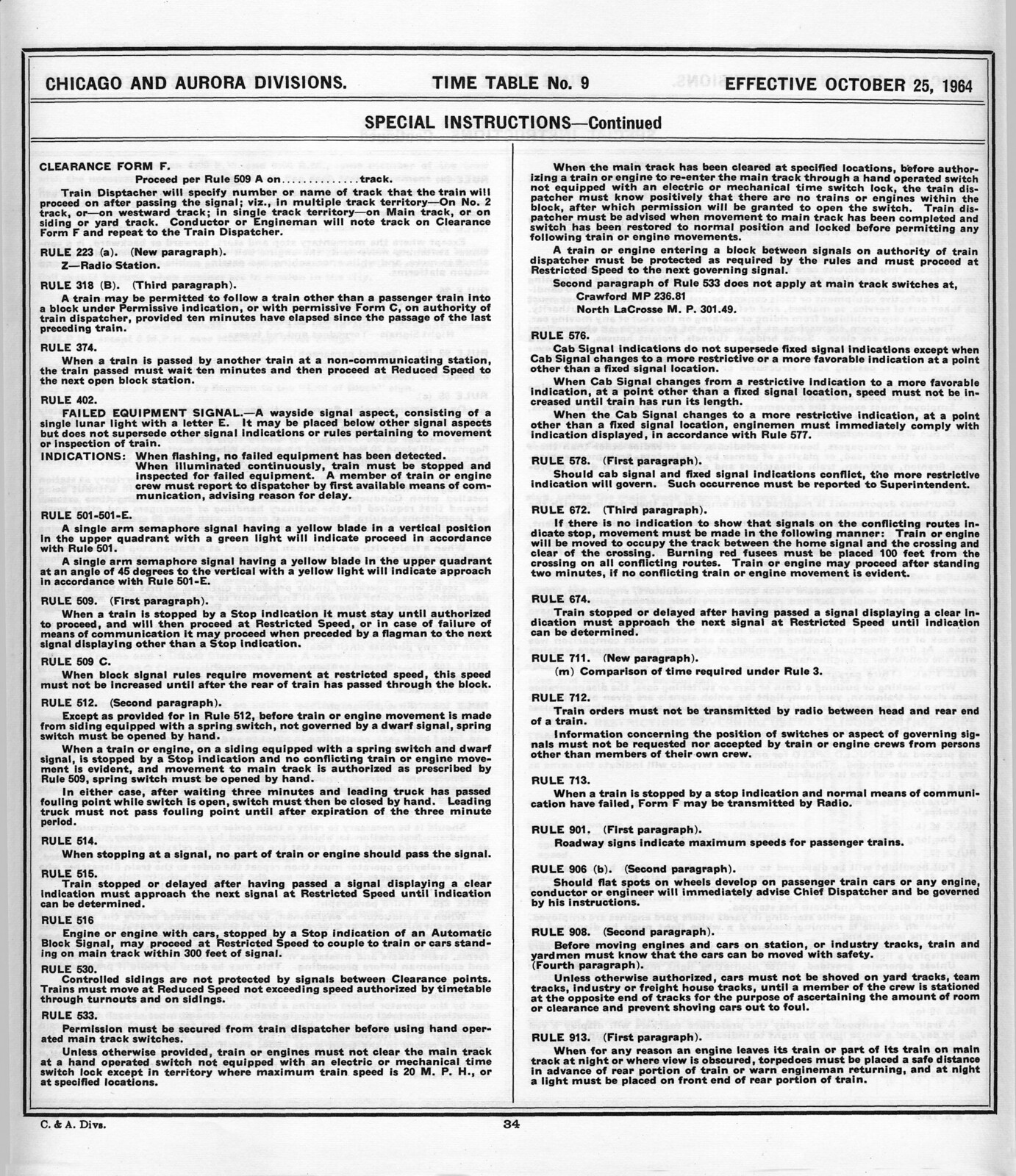The image is a vertically oriented, rectangular page from a business document or possibly an old timetable. It features two columns of very fine print text. At the top of the page, a header bar indicates "Chicago and Aurora Divisions" and "Timetable Number 9," which is effective as of October 25, 1964. Below this, the text reads "Special Instructions - Continued," signaling that the information carries over from a previous page. The lengthy text within the columns seems to detail various rules and instructions, such as rules 223, 318, 374, 908, and 913. It's filled with detailed guidelines, possibly related to operational or legal protocols. The page number, located at the bottom, is 34. The entire document is printed in black on white paper, contributing to its formal and detailed appearance.